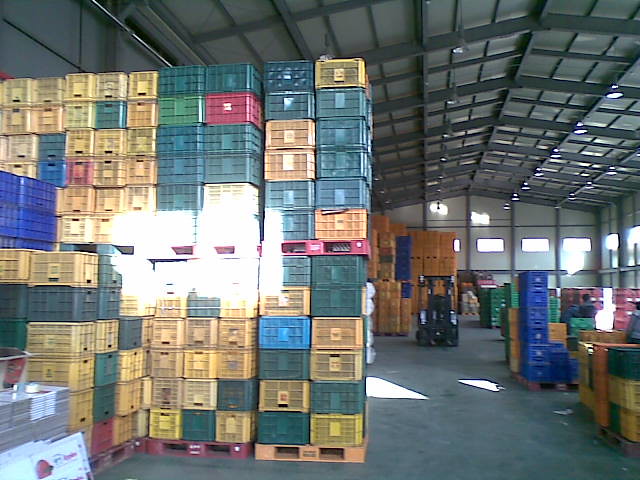The image captures a brightly lit, expansive storage warehouse with a high, peaked roof featuring a grid-like metal rafters structure. Rows of identical lights are suspended from the ceiling, casting an even illumination throughout the large room. The ground is dark gray concrete, adding to the industrial feel of the space.

In the foreground, there is a towering wall of colorful plastic crates stacked nearly from floor to ceiling. These crates, arranged on single layers of wooden pallets, are varied in color—predominantly green, yellow, red, and blue. Some pallets are distinctly red or orange. 

Midway into the warehouse, slightly blurred due to lighting and focus, there is a black forklift truck barely visible with just the tires and some structure discernible. Additional stacks of crates, mainly orange and blue, can be spotted towards the background on both sides of the aisle, creating a colorful landscape of organized storage. The warehouse feels cluttered but structured, showcasing the wide variety of goods stored within it.